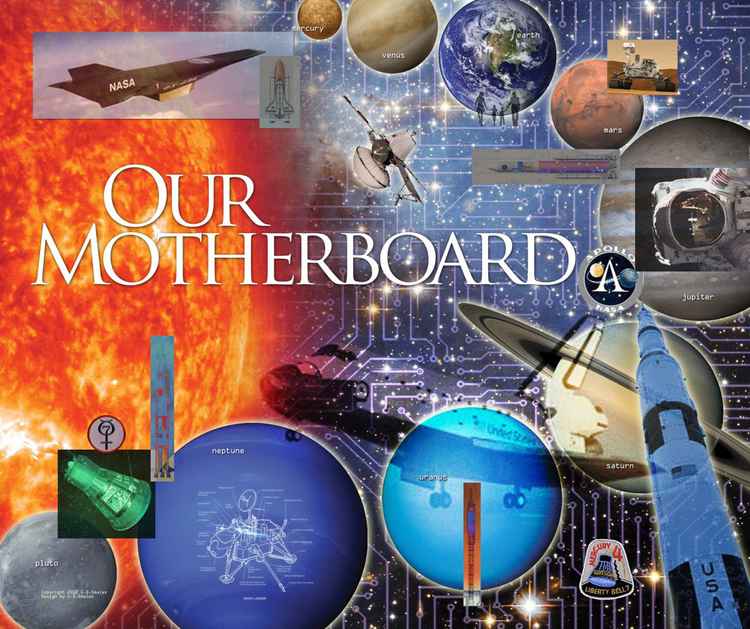The image titled "Our Motherboard" prominently features the text "Our Motherboard" slightly to the left of center in white letters. This visually striking montage showcases a blend of American military and space vehicles, equipment, and technology, creating a smorgasbord of aeronautics and computer imagery. Central to the piece is a black NASA plane, specifically the NASA X-43 hypersonic unmanned craft, located in the upper left corner. Adjacent to it is the iconic Voyager 2 space shuttle.

The image includes various historical spacecraft: the Mercury capsule on the lower left corner, the Apollo mission equipment on the lower right, and the Viking probe from 1976. Above these, an astronaut's head and figures such as the Perseverance rover find their place amidst the composition. The Artemis rocket is also discernible.

The background is a vibrant contrast of colors, with the left side dominated by an orange hue due to an orange planet (possibly Mars), while the right side is blue, exhibiting a detailed motherboard texture complete with interconnected white and silver wires, aligning with the title's theme.

Additionally, the solar system's nine planets are meticulously illustrated, spiraling from the top left of the image around to the bottom left. The celestial bodies are arranged in order: Mercury, Venus, Earth, Mars, Jupiter (which is superimposed over the motherboard texture), Saturn, Uranus, Neptune, and Pluto. Notable superimpositions include a rocket over Uranus and the Viking probe on Neptune, enriching the image's intricate detailing and emphasizing its dedication to NASA's technological advancements.